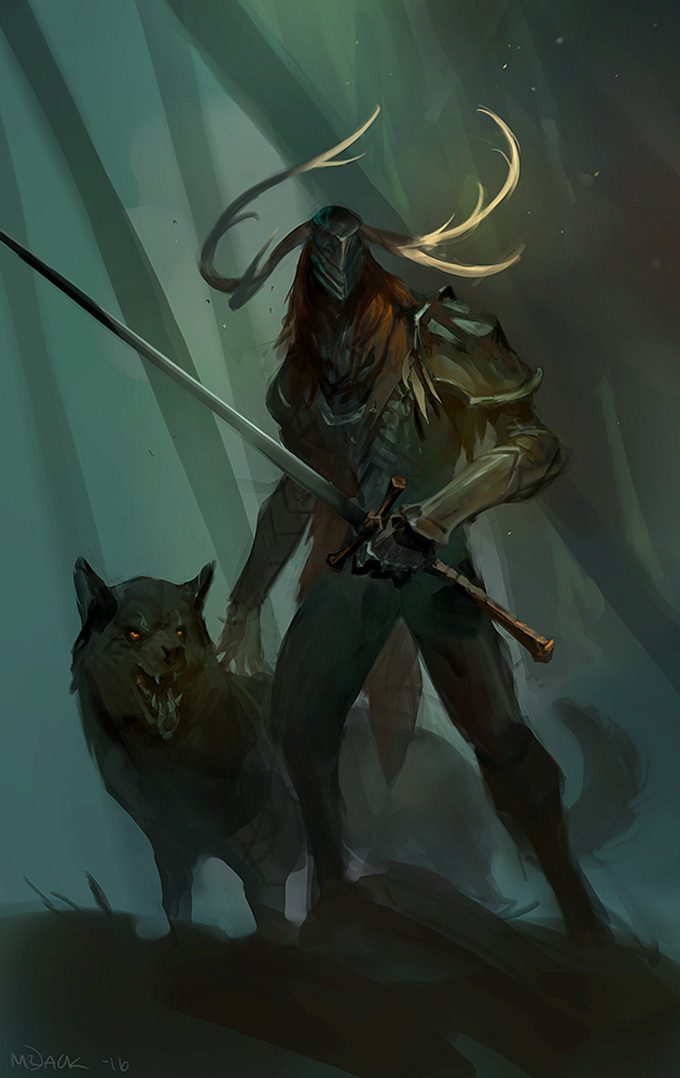In this detailed artistic image, the lower background is a dark gray shade, resembling ground cover or grass. As the scene ascends, it transitions into a blend of teal and gray hues, evoking the impression of tree stems and branches angled upwards. Highlighted with splashes of green and gray, the intricate backdrop adds to the surreal atmosphere.

Centrally, a striking creature commands attention. It sports elaborate yellow antlers and wears a gray metal helmet that conceals its face. Flowing orange hair cascades down its shoulders, contrasting with the creature's formidable gray metal body armor. It brandishes a long silver sword with a striking red handle, enhancing its imposing presence. The creature’s legs are equally armored in gray.

Adding to the mystical scene, a gray wolf with vivid orange eyes, white sharp teeth, and pointy ears stands beside the creature, emphasizing the image's fantastical and adventurous essence.